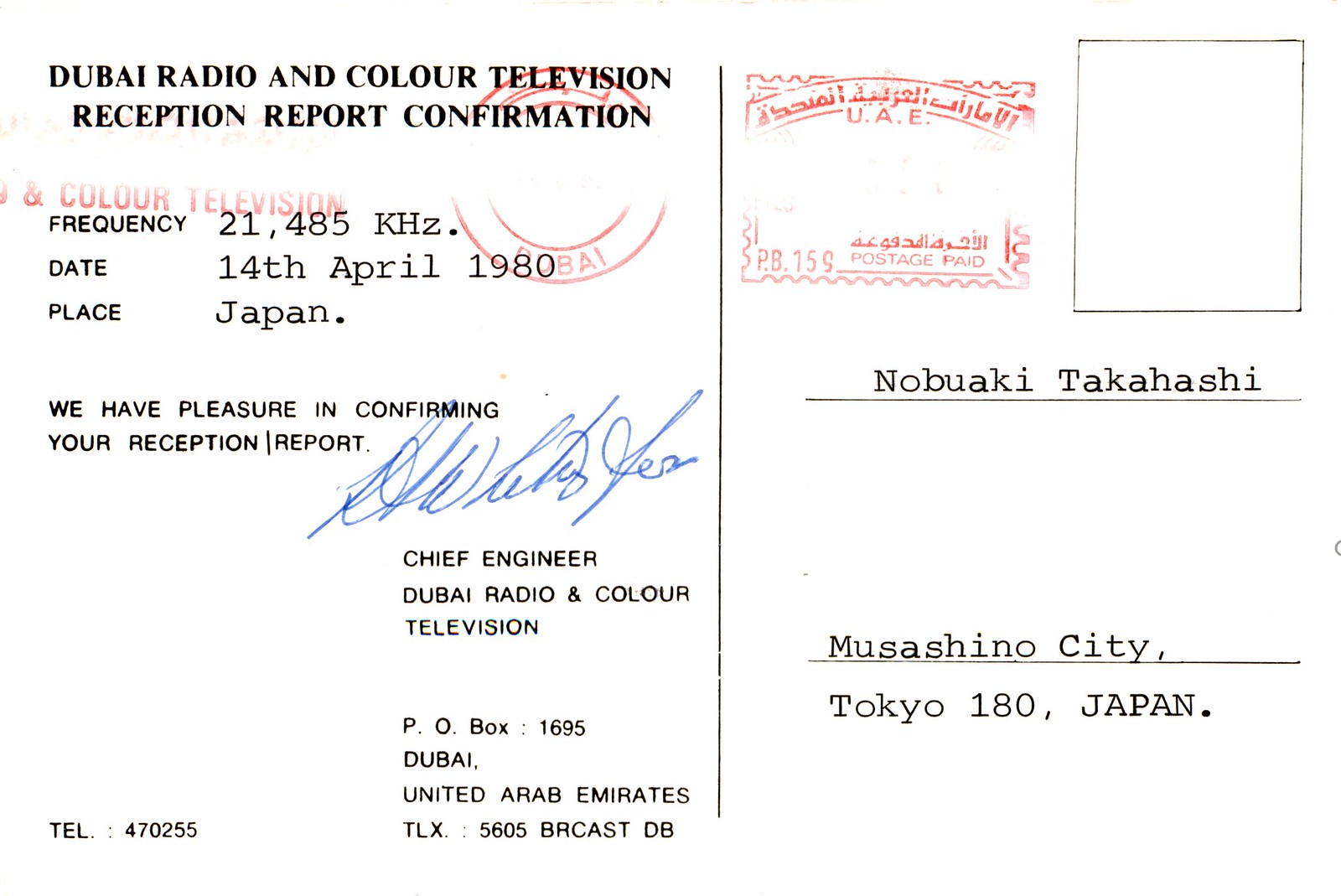This image is of a wide, rectangular postcard with a slightly off-white background. On the left side, the bold, black, all-capital letters read "DUBAI RADIO AND COLOR TELEVISION RECEPTION REPORT CONFIRMATION." At the top left corner, there's a red circular stamp, albeit slightly faded, overlapping part of the heading. Below this, the text reads: "Frequency: 21,485 KHz, Date: 14 April 1980, Place: Japan." Following that is the phrase, "We have pleasure in confirming your reception report." Further down, a blue pen signature is present, accompanied by the title "Chief Engineer, Dubai Radio and Color Television." The bottom left corner contains a telephone number: 4070255.

On the right side of the postcard, there's an underlined name, "Nobuaki Takahashi," followed by the address "Musashino City, Tokyo 180, Japan." A blank rectangular box, likely intended for a postal stamp, is located at the top right. Just to its left is another red circular stamp that has a logo in Urdu, the word "Nishwad," and notes "UAE" along with a postage paid mark mentioning "P.B. 159" and some Urdu script. At the very bottom on the right side, additional details read "P.O. Box 1695, Dubai United Arab Emirates" and "TLX 5605 BR Cast in DB."

This detailed depiction of the postcard emphasizes both textual content and layout, providing significant insight into its design and elements.